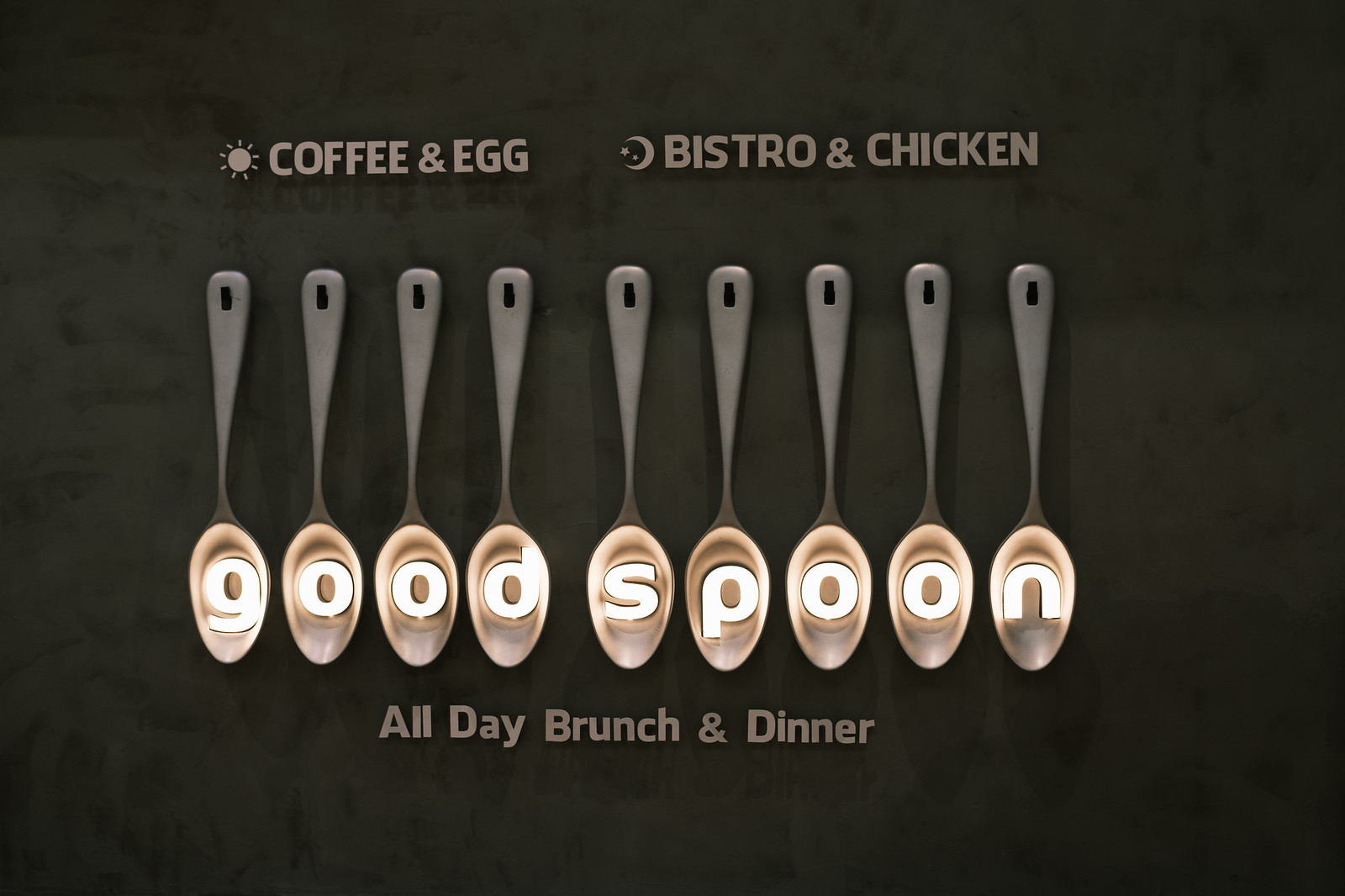This image appears to be a photograph, possibly of a restaurant sign or menu, against a dark, blackish-gray background. The aspect ratio is rectangular, being wider than it is tall. At the top of the image, in gray letters, is a detailing that includes a small sun symbol followed by the words "coffee & egg," and next to it, a crescent moon with two stars alongside the words "bistro & chicken." Below these elements, situated in the center of the image, are five silver-gray spoons, arranged horizontally and hanging from their handles, each of which features a black dot, potentially a hole. Within the bowls of the spoons are white letters that spell out "GOOD SPOON." Lastly, at the bottom of the image, in gray lettering, it states "all day brunch & dinner." This thorough detailing lends a sense of artistry to the image, highlighting both individual and combined elements to imply it represents a restaurant branding.